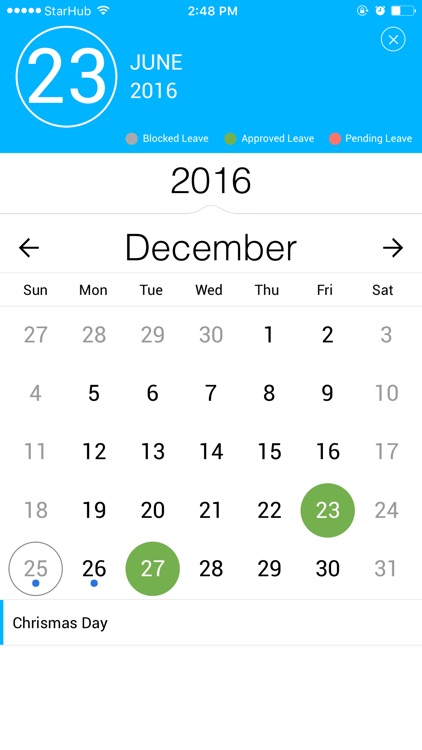The image displays a digital calendar for December 2016. The user is currently viewing the calendar via a calendar app, and it is noted that today is the 23rd of June, 2016. The calendar highlights events on the 25th and 26th of December, though these might be default entries within the app. Specific days, such as the 23rd and 27th, are highlighted, suggesting that the user may intend to add events to these dates.

At the top of the calendar interface, there is a legend using color-coded categories: brown indicates "blocked leave," green signifies "approved leave," and red denotes "pending leave." This suggests the calendar is used for managing employee leave, indicating when staff are permitted or restricted from taking time off. Based on the current entries, it appears the individual has approved leave scheduled for the 23rd and 27th of December.